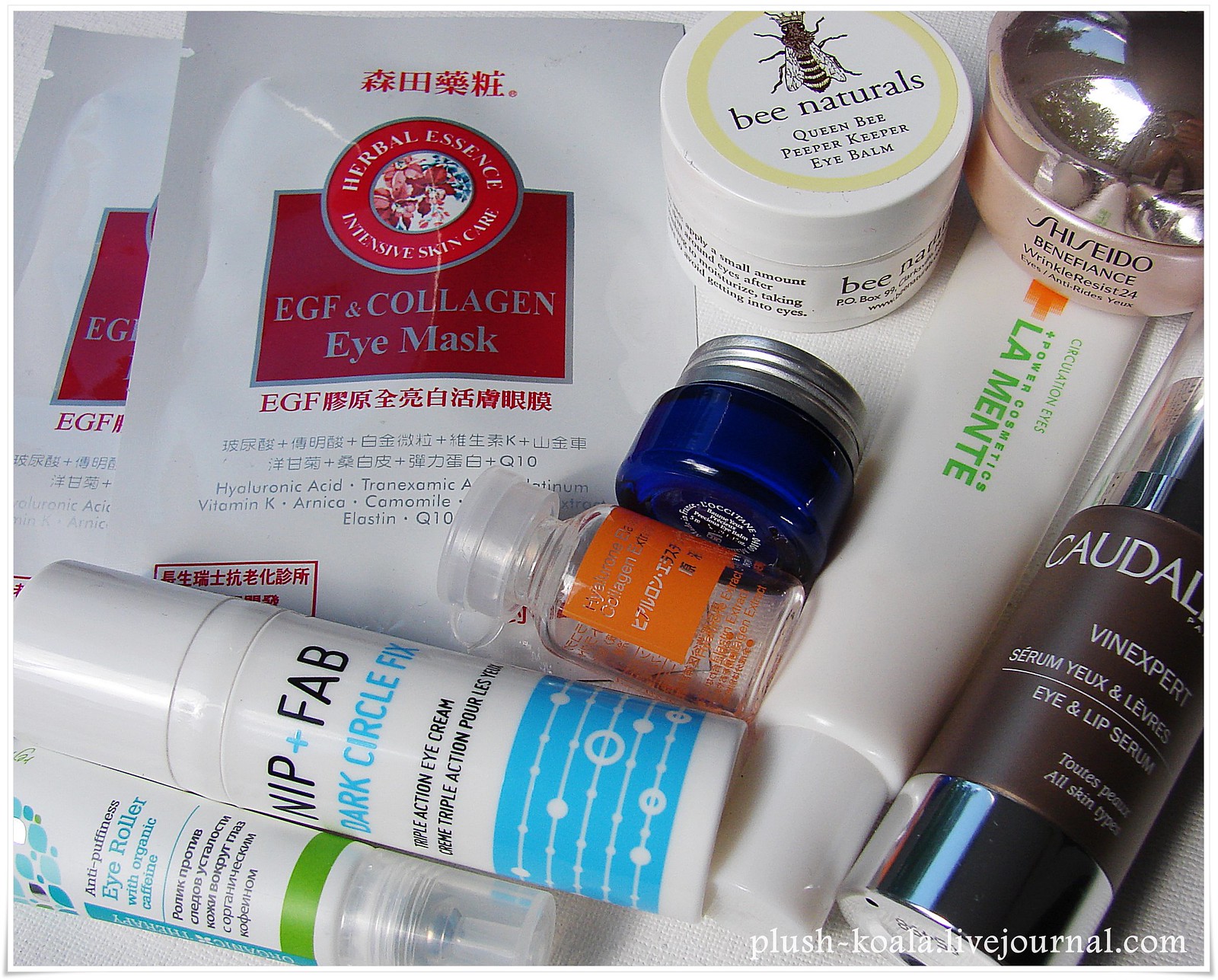This detailed image portrays a collection of ten curated skincare items arranged thoughtfully. At the bottom right, the image is credited to plush-koala.livejournal.com. The collection features a variety of eye care products from different brands, with some text in Eastern languages and English mingled together.

On the top left, two distinct packs of EGF and Collagen Eye Masks are visible, bearing an "Herbal Essence" logo and additional skincare branding. To the right, there is a Nip and Fab Dark Circle Fix, Triple Action Cream, presented in a sleek white vial with a blue band and dotted design on the bottom.

In the bottom left corner, an Anti-Puffiness Eye Roller infused with Organic Caffeine features a blue strip along its side and a green strip on the bottom, complete with a push sprayer cap. Moving to the top right, a small jar marked with a bee logo reads "Bee Naturals, Queen Bee, Peeper Keeper Eyebalm."

Adjacent to it, on the bottom right section, a tube of Shiseido Benefiance WrinkleResist24 Eye Cream is partly visible, labeled as a potent anti-aging solution. Nearby, a product named Circulation Eyes from Power Cosmetics, labeled "La Mente" in green text on a white tube, adds to the eclectic mix.

Completing the set is a brown vial capped in silver, known as Caudalie Vine[Activ] Eye and Lip Serum, prominently annotated as a rejuvenating treatment. This well-rounded selection reflects a commitment to comprehensive eye skincare, blending various global influences and specialized formulas.